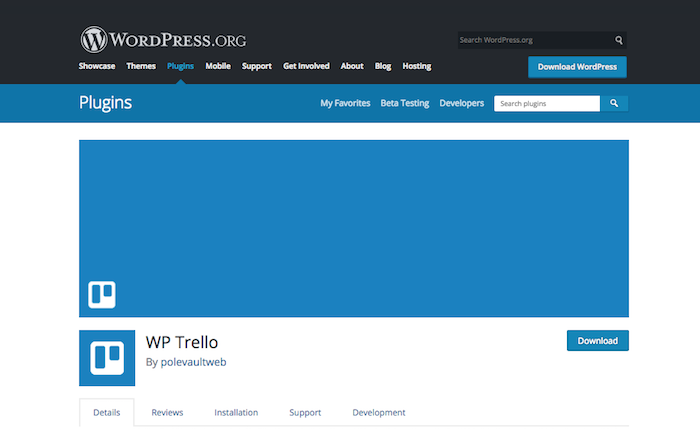The image showcases the WordPress.org website interface. At the top of the screen, the WordPress.org logo is displayed prominently. To the right of the logo is a search bar. Below this menu, categories are listed horizontally from left to right: Showcase, Themes, Plugins (highlighted in blue as the selected option), Mobile, Support, Get Involved, About, Blog, and Hosting. 

On the right side, a notable blue button labeled "Download WordPress" stands out. Below that, the "Plugins" section is opened, revealing three subcategories: My Favorites, Beta Testing, and Developers. Another search bar appears to the right, characterized by a white input area and a blue search button.

A popup is visible below this section, primarily set against a background of a large blue rectangle with a white square at the bottom left corner. Within the white square, the text "WP Trello" is displayed alongside a blue square with the text "Pole Vault Web". To the right, a small blue rectangle marked "Download" is present. 

Five tabs are lined up below this popup, each described as follows from left to right: Details, Reviews, Installation, Support, and Development. The entire interface maintains a clean white background, ensuring readability and organization.